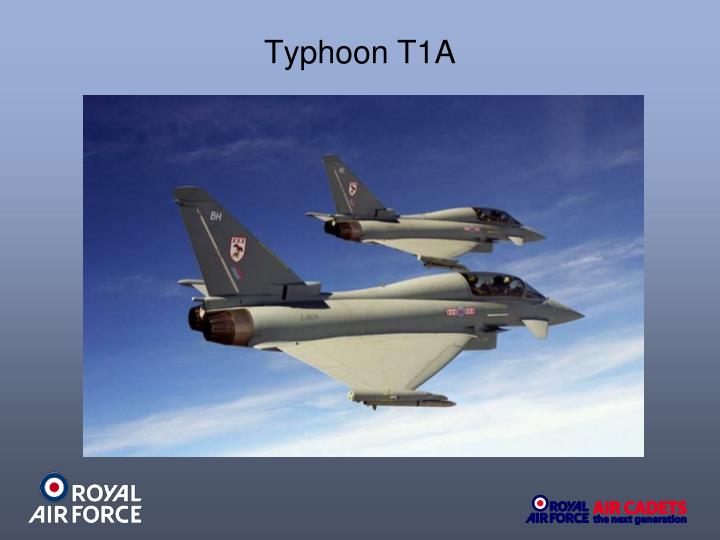The poster features an RAF scene within a thick, wide, light blue frame that transitions to a darker blue at the bottom. Dominating the composition are two Royal Air Force Typhoon T1A jets flying in formation towards the right against a vivid blue sky, subtly transitioning to a darker shade on the left and lightening towards the bottom right, where thin, white clouds appear. The jets themselves are predominantly grey with red markings: notably, a shield with a red winged bird on their rudders and red accents beneath the cockpit, which is a dark translucent grey. The larger jet in the foreground starkly contrasts with the smaller one receding into the background. Prominently printed at the top of the image is "Typhoon T1A" in black lettering. The bottom left corner features the RAF logo—a circle with a blue edge and a red dot in the center—with the text "Royal Air Force" adjacent. The bottom right corner repeats "Royal Air Force" in blue lettering and includes the phrase “Air Cadets” in red, underscored by the slogan "the next generation" in blue.